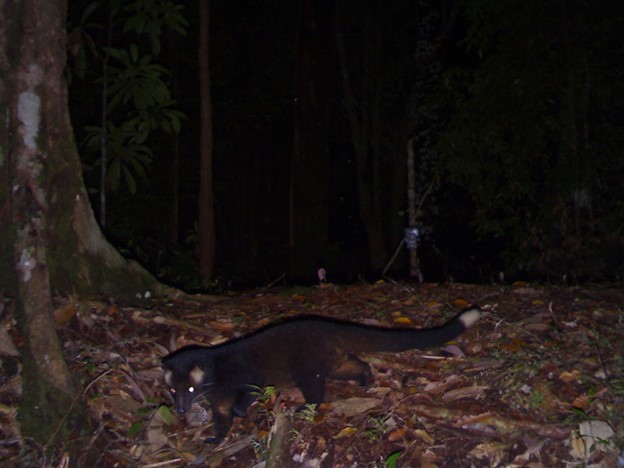In this nighttime outdoor photograph, we see a small, four-legged animal captured by a trail camera in a dense, wooded setting. The scene is illuminated by the camera's flash, revealing a dark environment with multiple trees and a forest floor littered with fallen brown leaves, sticks, twigs, roots, pine cones, and small green sprouts. Prominently in the center, the animal—a black-furred rodent or marsupial with distinctive white patches above its eyes, on its ears, and at the tip of its long tail—is moving towards the left side of the image. The creature's eyes glow due to the camera's flash, and its pointed face and short muzzle are turned towards the camera, capturing a moment of surprise. On the left side, a large, moss-covered tree trunk stands close to the camera, surrounded by green leaves. In the background, the darkness renders most details indistinct, but amid the trees, a reflective object can be seen on one of the trunks. The surreal quality of the photograph is heightened by what appears to be the faint outline of a human figure standing in the background, their face partially visible.